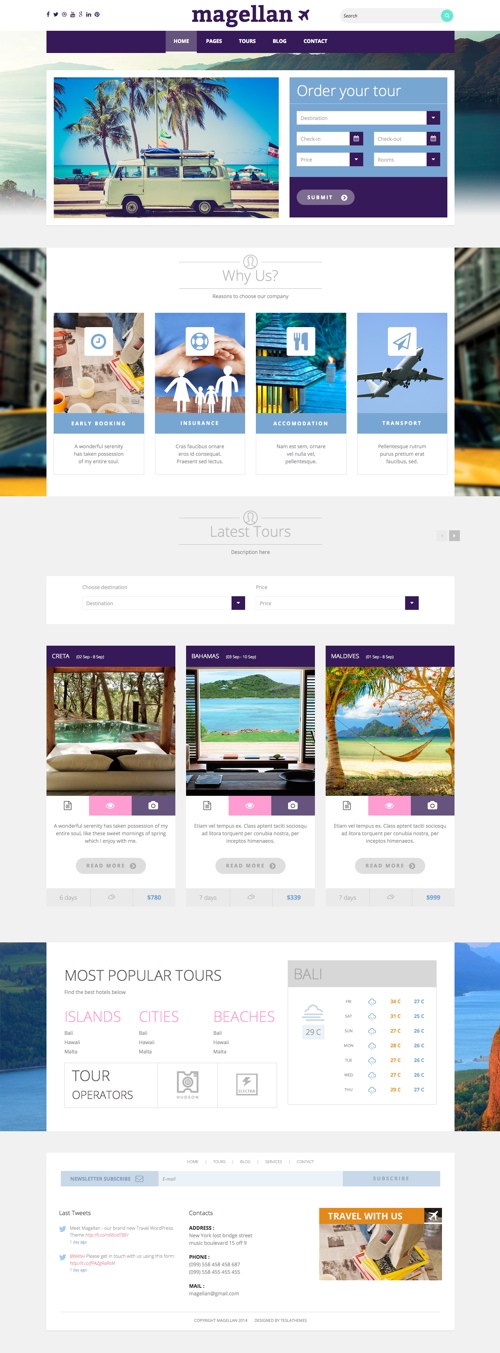This image is a screenshot of a mobile website designed for travel booking, viewed in portrait orientation. The screenshot is significantly taller than it is wide, providing a comprehensive view of various sections of the website.

At the top of the image, there is a white border featuring centered, purple text that reads "Magellan," accompanied by a graphic of an airplane ascending to the right, located to the right of the word "Magellan." On the far left of this border are small icons that appear to be social media links, though the details are too minute to identify precisely. On the far right, there is a grey search bubble with a green circular icon at its end, containing a white magnifying glass, followed by some unreadable black text.

Below this top section, a purple rectangular navigation bar spans the width of the screen, displaying clickable options in white text. The first option is highlighted and features a subtle shadow effect, suggesting it is the currently selected or active option.

The main content begins with an image of a classic Volkswagen Beetle Van or Volkswagen Van parked beside a beach, complete with a palm tree. Adjacent to this image, on the right, is a blue box containing the text "Order Your Tour," along with white boxes with purple icons that allow user input.

Beneath this section is a white area with the heading "Why Us," followed by four selectable options related to food and other activities. Below this are three more boxes outlined in purple, displaying images of attractive outdoor settings. This section concludes with a suggestion for the most popular tours available on the website.